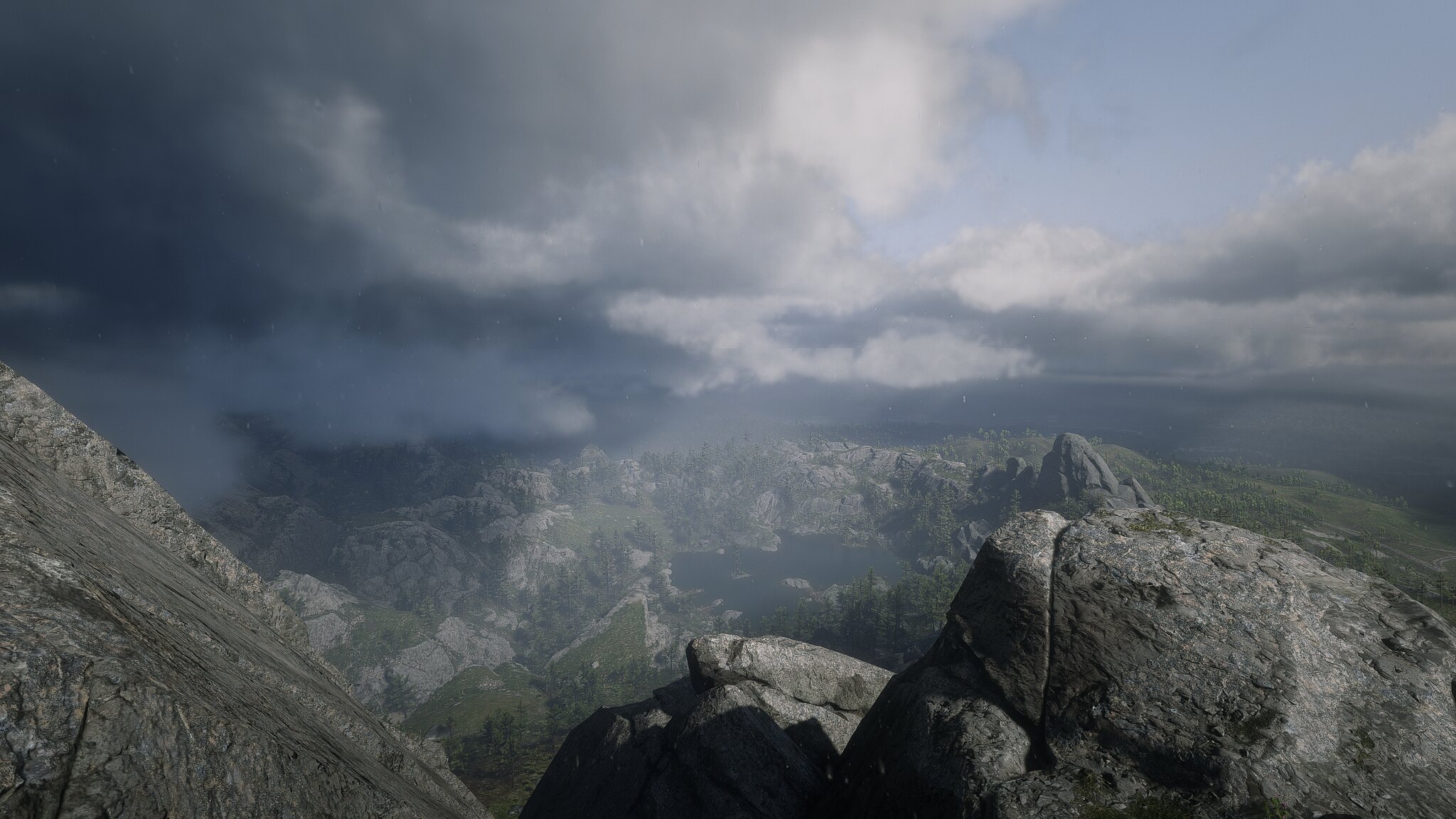This photo captures a dramatic mountain landscape from an elevated vantage point. In the foreground, three prominent rocks—two flanking the left and right sides and one positioned in the center—command attention. Far below, patches of green grass frame the rugged terrain, while a possible body of water glimmers amidst the rocky expanse. Above, a canopy of clouds dominates the sky, with layers ranging from dark gray storm clouds to lighter gray and even some white patches, allowing glimpses of a pale blue sky to peek through. The scene is further enriched by the interplay of colors and textures: the storm clouds, gray and varied in shade, juxtapose against the lighter, almost ethereal gray of the rocks, and the vibrant green of the surrounding grass provides a striking contrast. The entire view is encircled by a sense of grandeur and isolation, enhanced by the cloudy atmosphere that casts a serene yet tempestuous mood over the landscape.